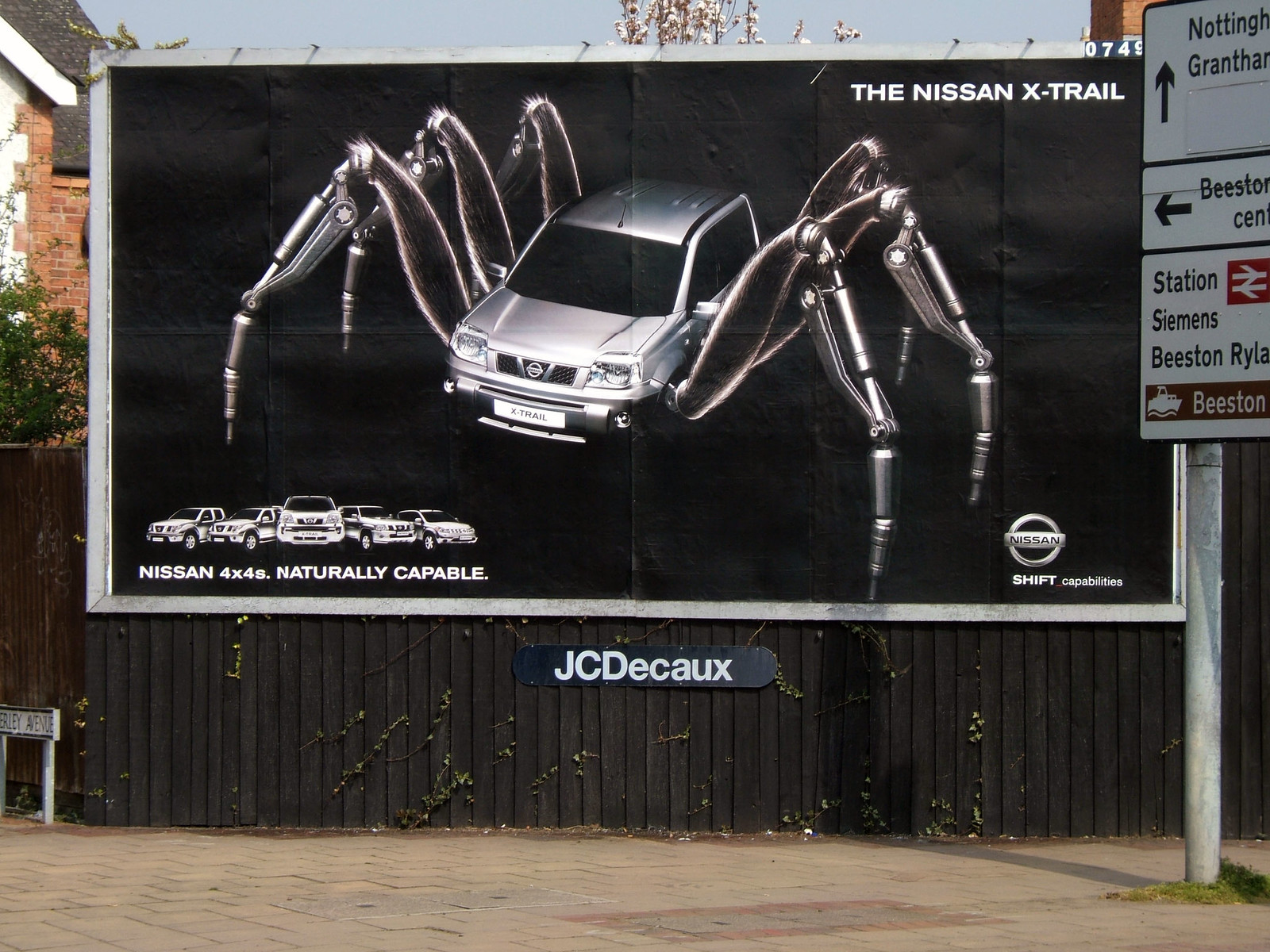The image captures a photograph of a billboard prominently centered and slightly elevated above a dark brown wooden fence with a scattering of leaves possibly from a nearby bush. This rectangular billboard is bordered in silver and features a predominantly black background. At the center of the advertisement is a silver Nissan X-Trail SUV, whose windows are completely blacked out. The vehicle is depicted with six mechanical, spider-like legs—three on each side—constructed from steel and hydraulics, giving the SUV an insect-like or crab-like appearance. 

In the upper right corner of the billboard, the text "The Nissan X-Trail" is displayed in white. At the bottom left corner, there is a small image showing a lineup of five various Nissan vehicles with the caption "Nissan 4x4s, naturally capable" beneath it. In the lower right corner, the Nissan emblem is showcased, accompanied by the slogan "Shift Capabilities" below it.

The setting around the billboard includes a black fence with the text "J-C-D-E-C-A-U-X" in white against a black background located at its center, directly beneath the ad. The background features hints of a blue-gray sky and a partially visible brick house to the left of the photograph. On the far right of the image, a street sign is partially visible, indicating the names "Nottingham" and "Grantham." The foreground includes a light brown brick sidewalk.